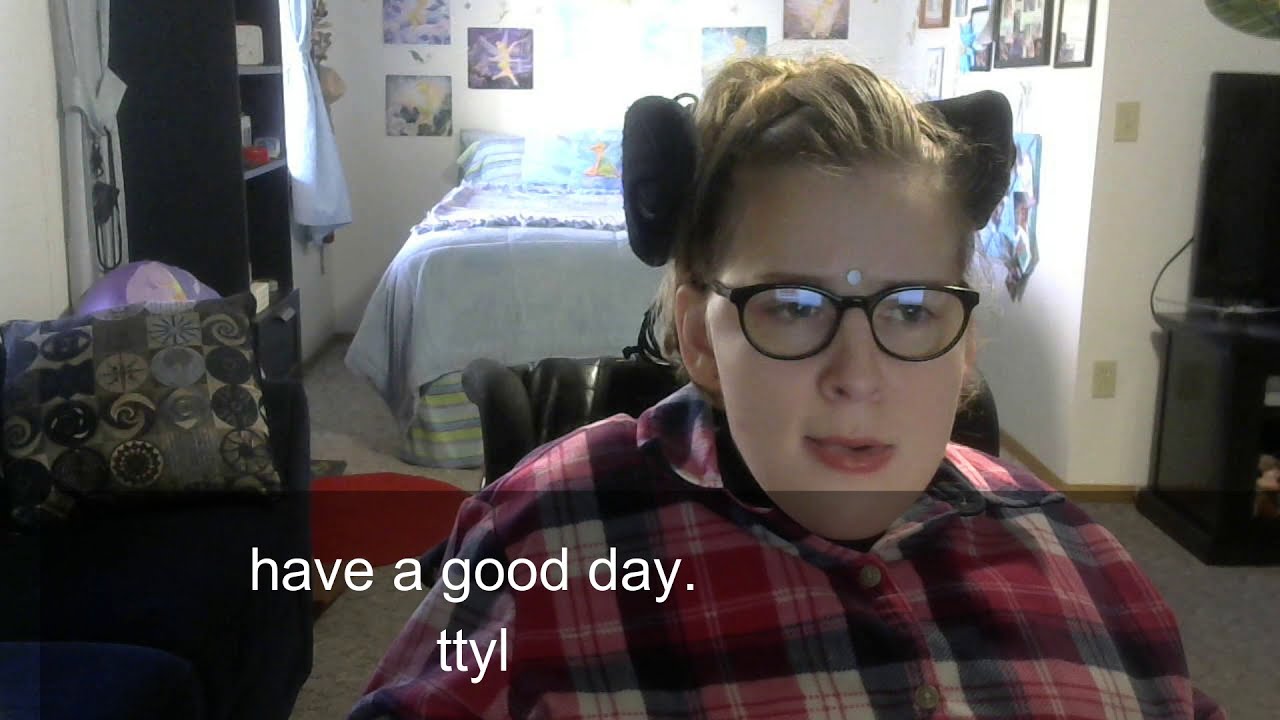The photograph is a color landscape image depicting a young girl, approximately 12 or 13 years old, taking a selfie in her bedroom. She is positioned slightly to the right of center and is wearing black glasses and a red and blue plaid shirt. Her blonde hair is short, and she has black headphones propped on top of her head, along with a small white sticker circle between her eyebrows. Behind her, a black headrest is visible, indicating she might be sitting in a wheelchair. Her bedroom walls are white and adorned with framed artwork and posters. The background features a made bed with a white cover, a blue couch with a gray geometric pillow, a black dresser, and bookshelves on either side. Superimposed at the bottom of the image, in white text, is the message: "Have a good day. TTYL." She appears to be looking directly at a screen, capturing a moment of casual interaction in a cozy and organized space.